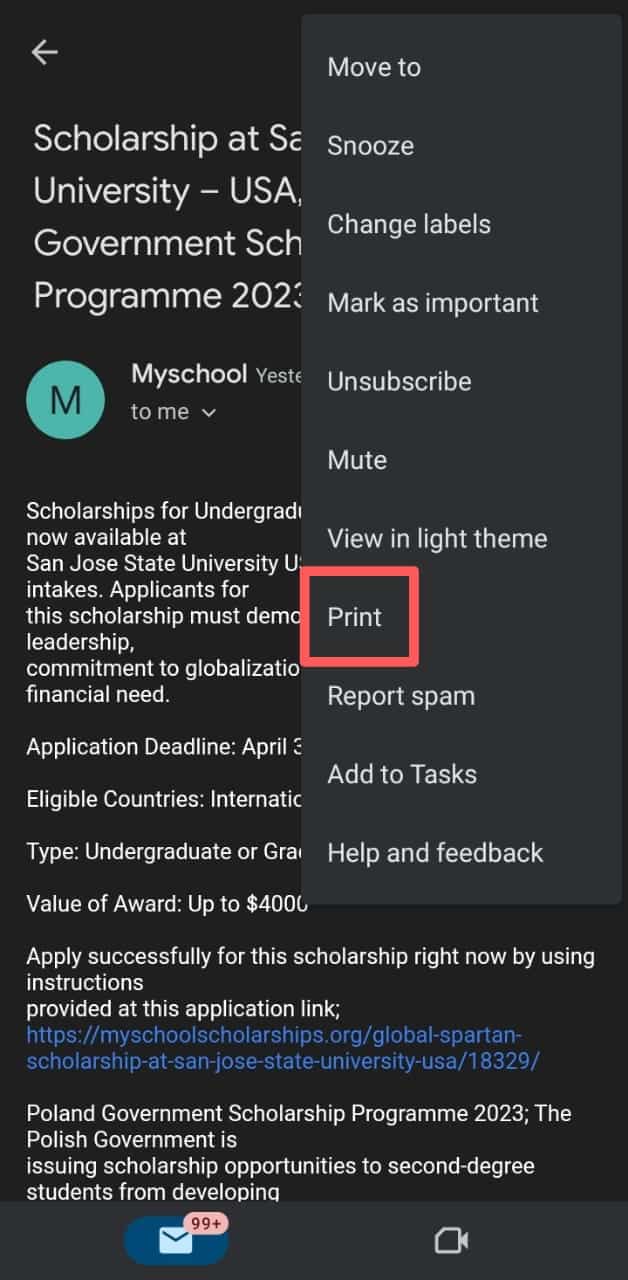This image appears to be a screenshot taken from a smartphone. It features a vertical rectangle with a black background and white text in the center. At the top of the image, there's a pop-up box over the background screen, also predominantly black with white text.

On the left side of the main text area, you can discern some keywords indicating a scholarship opportunity at "San Jose State University," associated with a "USA government program" for the year 2023. Nearby, there is a blue circle containing the letter "M" and the label "My School." Below this, the text announces that undergraduate scholarships are now available for applicants at San Jose State University.

The text specifies that applicants for this scholarship must demonstrate leadership, show a commitment to globalization, and have financial need. It also mentions an application deadline, urging potential candidates to apply successfully by following the provided instructions, which are accessible via a blue hyperlink.

On the right side of the image, there's an additional pop-up in gray with white text. It appears that the user has clicked a print option, indicated by the word "Print" enclosed in a large red rectangle.